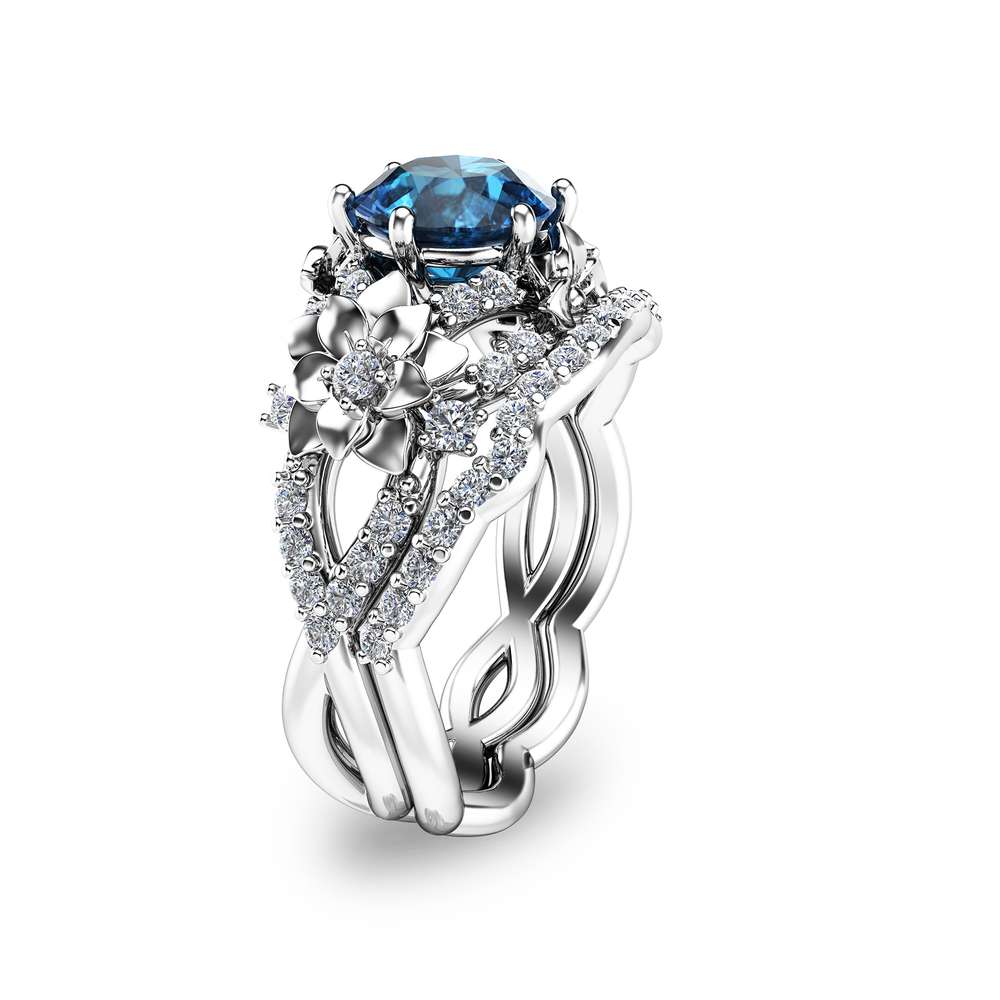The image showcases a stunning silver ring set against a completely white background, highlighting its intricate design. Positioned at the center, the ring stands on its end, tilted slightly to the left, revealing both its interior and exterior details. The band is composed of three intertwined silver strands, creating a braided, figure-eight pattern that lends an air of elegance.

Dominating the ring is a large, eye-catching blue stone, securely held in place by seven prongs. Surrounding the blue stone, there are numerous small diamonds adorning the top bands of the ring, adding a touch of sparkling brilliance. On the visible side of the ring, a silver flower embellishment with six inner petals and five outer petals is prominently featured, centered by a radiant diamond. The ring's meticulous craftsmanship and the combination of silver, diamonds, and the vibrant blue stone make it an exquisite piece of jewelry.